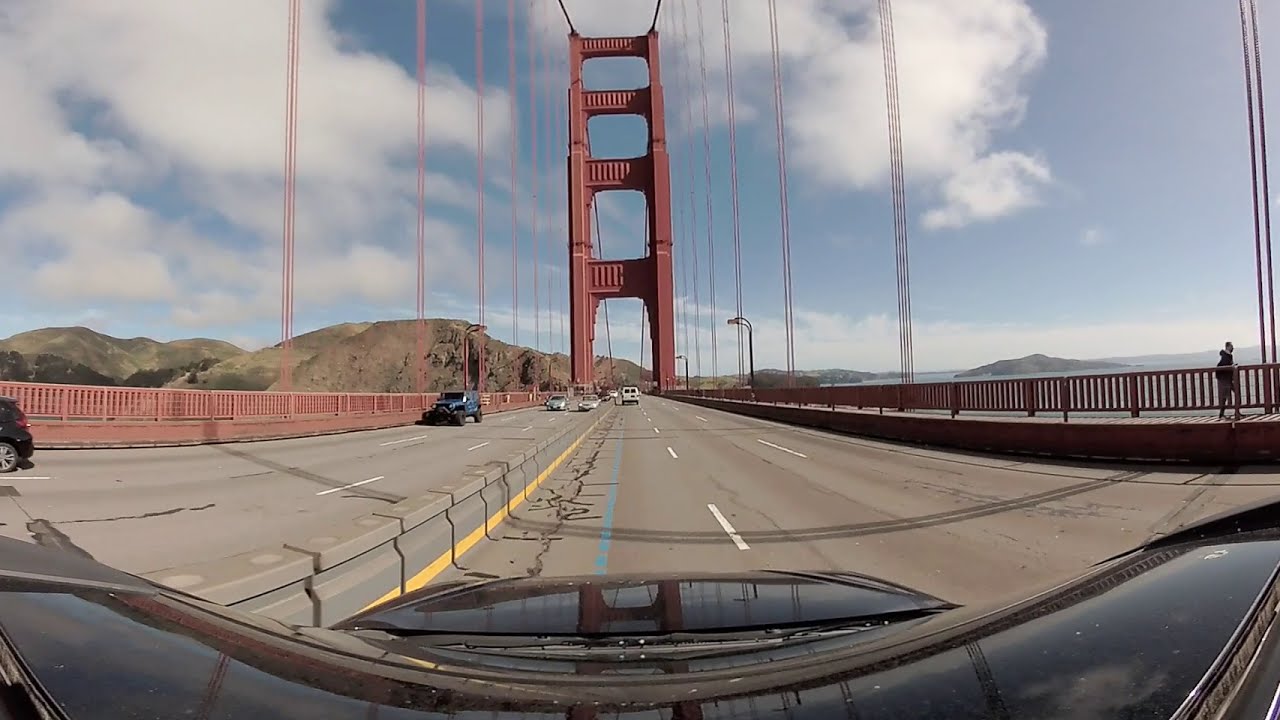This image is a photograph taken from the windshield of a car driving across the iconic Golden Gate Bridge. The bridge, known for its striking reddish-orange color, features towering cables and matching walls and ledges. The road surface is light gray with dashed white lines marking the lanes, and a solid gray jersey wall divides the opposing directions of traffic. There are six lanes in total, three for each direction of travel. On the right side of the image, we see vehicles moving forward, while on the left, cars are headed towards the viewer, including a notable blue jeep and several silver cars.

In the background, brownish-green mountains rise up under a sky filled with white, puffy clouds, casting a serene contrast to the bustling bridge. The sky itself is a soft blue, hinting at a sunny day. The photograph captures a dynamic moment on the bridge, emphasizing its grand scale and the mix of pedestrian and vehicle traffic that it supports. The image slightly distorts towards the edges due to the lens, bending the view downward but adding a unique perspective to this iconic structure.